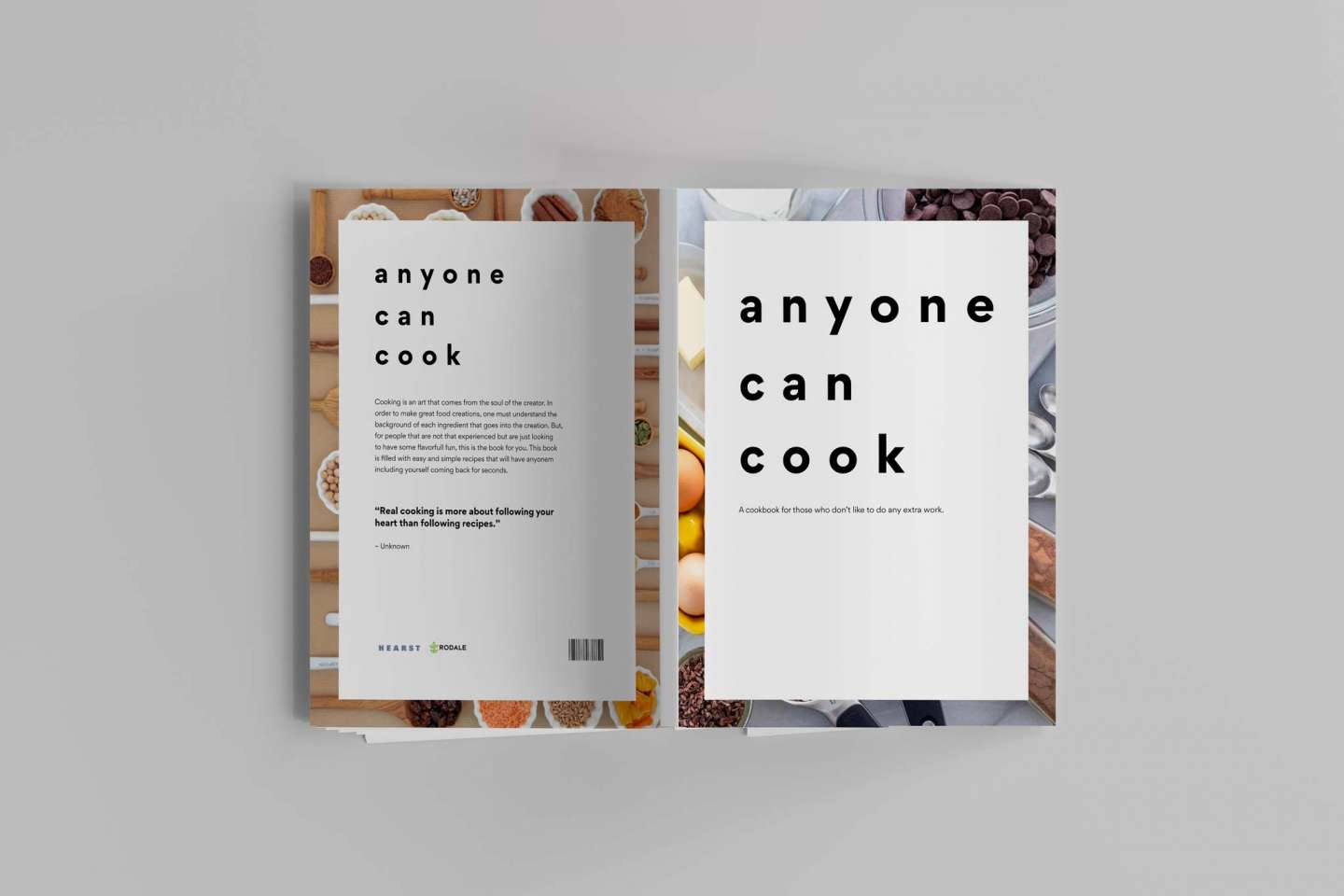The image shows a digital mock-up of the front and back cover of a cookbook titled "Anyone Can Cook." The book is displayed open and flat against a pale gray background, with both covers facing upwards. Dominating both covers is a large white rectangular box that takes up approximately 80% of the space. On the front cover, the title "Anyone Can Cook" is prominently displayed in a sans-serif, lowercase black font. The background behind this white box features a variety of cooking and baking items, including a bowl of chocolate chips, a measuring cup of milk, some butter, and several brown eggs in a yellow egg container, along with measuring spoons and utensils.

The back cover mirrors the front with the same white rectangular box and the title "Anyone Can Cook" in the same font. Below the title, there is a descriptive paragraph and a pull quote, accompanied by a UPC barcode. The background of the back cover also showcases various cooking items, such as wooden measuring spoons, spices, seeds in small white bowls, and possibly raisins in a measuring spoon. The overall mock-up clearly appears to be digital, accentuated by unnatural drop shadows and a few fake digitized pages poking out from the bottom back cover.